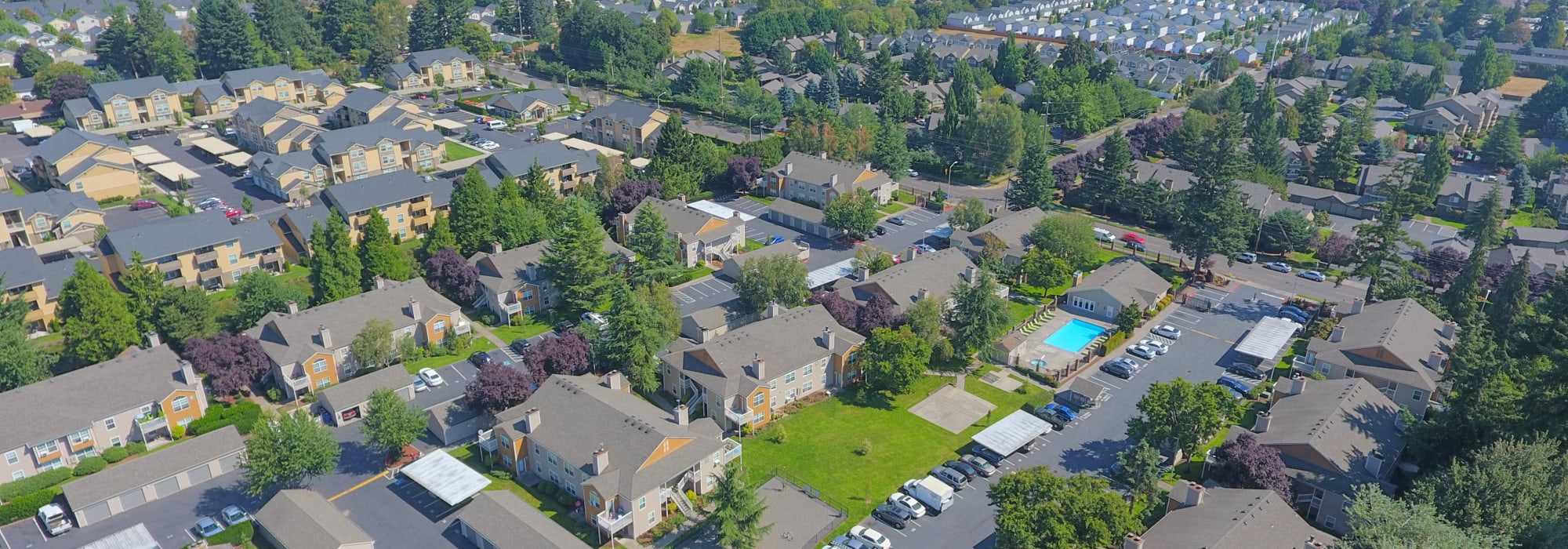The image depicts an aerial view of a suburban residential community filled with numerous apartment buildings characterized by gray roofs and a mix of yellow and gray façades. The buildings towards the top left corner showcase distinct yellowish walls with brown railing balconies, contrasting with the predominantly gray structures found elsewhere. Surrounding and interspersed among the buildings are a variety of green, leafy trees and a few purple-flowering trees, adding a vibrant touch to the scene under a sunny sky.

The bottom part of the image highlights a rectangular, light-blue swimming pool situated near a small, single-story house with a gray roof. Pool chairs are arranged around the pool area, and a line of parked cars is visible in front of it, indicating a nearby parking lot. The community is well-organized with neat rows of parking lots and roads, bordered by green areas and grassy patches. The image captures the serene and orderly nature of the suburb, reflecting a typical day in the neighborhood.